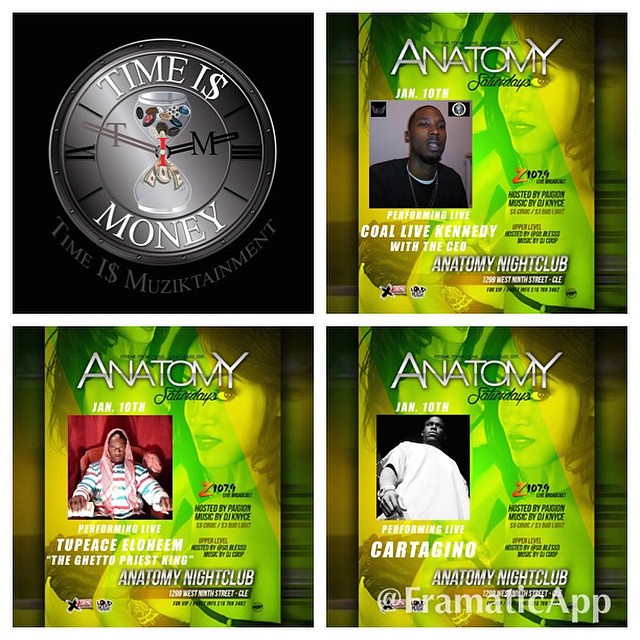The image is divided into four sections, each promoting a different event or performer at Anatomy Nightclub's "Anatomy Saturdays." 

In the top left section, a graphic displays a clock with the phrase "Time is Money" where the 'S' in 'is' is a dollar sign, and the word "Money" creatively incorporates various symbols and numerals around the clock face. An hourglass in the center of the clock is filled with chips and money, symbolizing the flow of time and wealth. The caption at the bottom of this section reads, "Time is Musictainment," emphasizing the theme of combining music and financial value.

The remaining three sections showcase promotional posters for Anatomy Nightclub. Each poster highlights a different performer, all of whom are black males:
1. Top right: A black man wearing a black shirt and necklace with the caption "Performing Live: CEO Paul Y. Kennedy."
2. Bottom left: A black man in a white, red, and blue striped shirt with a pink rag over his head, labeled "Performing Live: Two-Piece Elohim, the Ghetto Priest King."
3. Bottom right: A black and white image of a black man in a white shirt looking down, captioned "Performing Live: Cartagena."

Additionally, each poster features the text "Anatomy Saturdays" and provides event details such as the date (January 10th) and the hosting station or location at the bottom. The background of these posters includes images of women gazing seductively at the viewer, adding to the allure of the promotional materials. A subtle watermark is present at the bottom of the images, unifying the promotional theme.